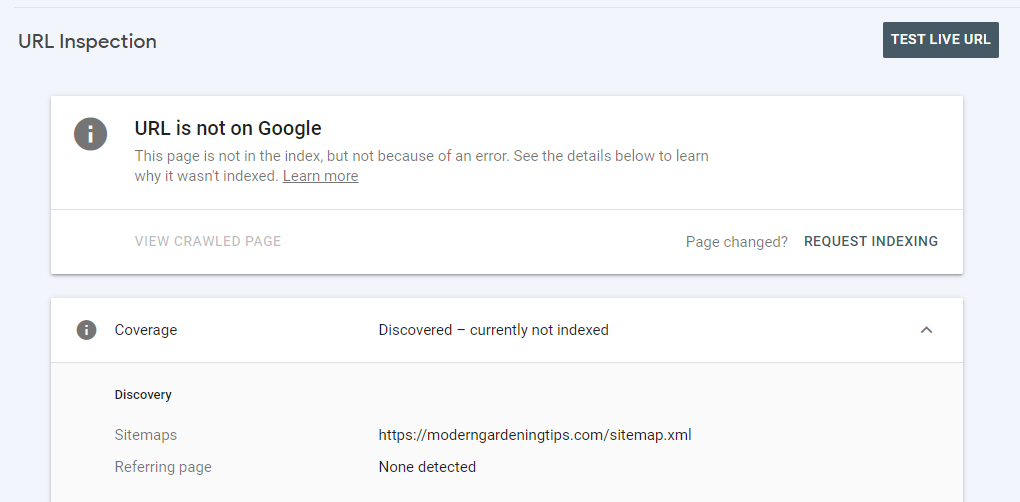This screenshot captures a URL inspection page from a website analytics tool. 

### Header Section:
- **Top Left Corner:** The title "URL Inspection" is prominently displayed in bold black letters.
- **Top Right Corner:** A black button with white text labeled "Test Live URL."

### Main Content:
- **Notification Area:** A white rectangular box contains an icon of a gray circle with a white eye. To its right, the message "URL is not on Google" appears in black text. Below this, an explanation reads, "This page is not in the index, but not because of an error. See the details below to learn why it wasn't indexed." An underlined "Learn more" link is also present.
  
### Details Section:
- **First Detail Block:**
  - **Left:** "View crawled page" in gray text.
  - **Right:** "Page change" and "Request indexing," both in gray text.

- **Second Detail Block:**
  - **Left:** Another white rectangular box contains a gray circle with a white eye icon.
  - **Right:** "Coverage" in black text. Below it, the status "Discovered - currently not indexed" in black text and an upward-facing arrow.

### Discovery Section:
- **Left:** The word "Discovery" in black text.
  - **Sub-item:** "Sitemaps" in gray text.
  - **Right:** "https://moderngardeningtips.com/sitemap.xml"
  
- **Referring Page:**
  - **Left:** "Referring page" in gray text.
  - **Right:** "None detected" in black text.